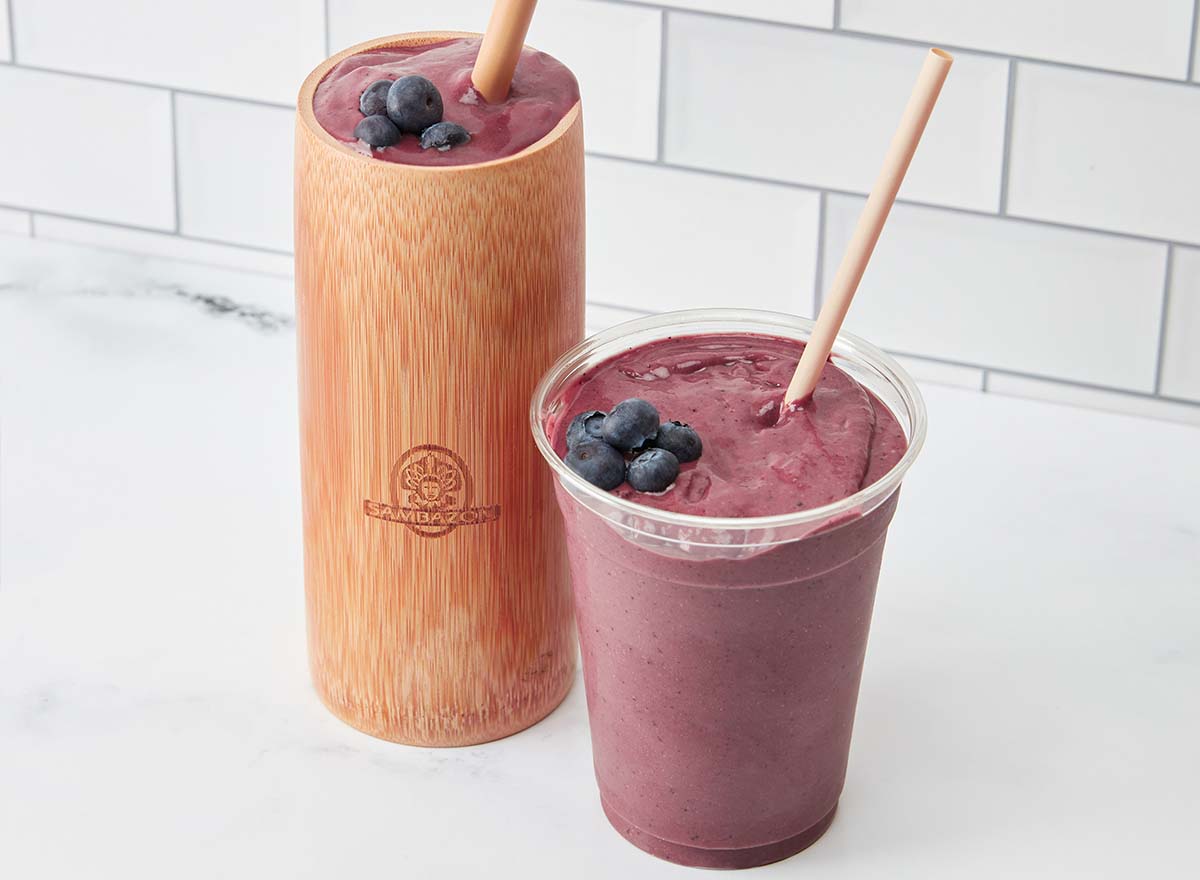This is a detailed photograph of two blueberry smoothies. The smoothie on the left is in a slightly taller, uniquely textured cup with an orange and tan, almost wooden-like appearance. This cup features a logo in brown that reads “Sambazon,” accompanied by an image of a small person with outstretched arms and a headdress with feathers of varying lengths. The right smoothie is housed in a clear plastic cup. Both purple-colored smoothies are topped with several blueberries, creating a visually appealing garnish. Each smoothie has a straw, with the cup on the left having a tan straw, while the right plastic cup features a clear plastic straw. The drinks are placed on a white and gray granite countertop, and the background reveals a white subway-tiled wall with gray accents, adding a clean and modern aesthetic to the image.